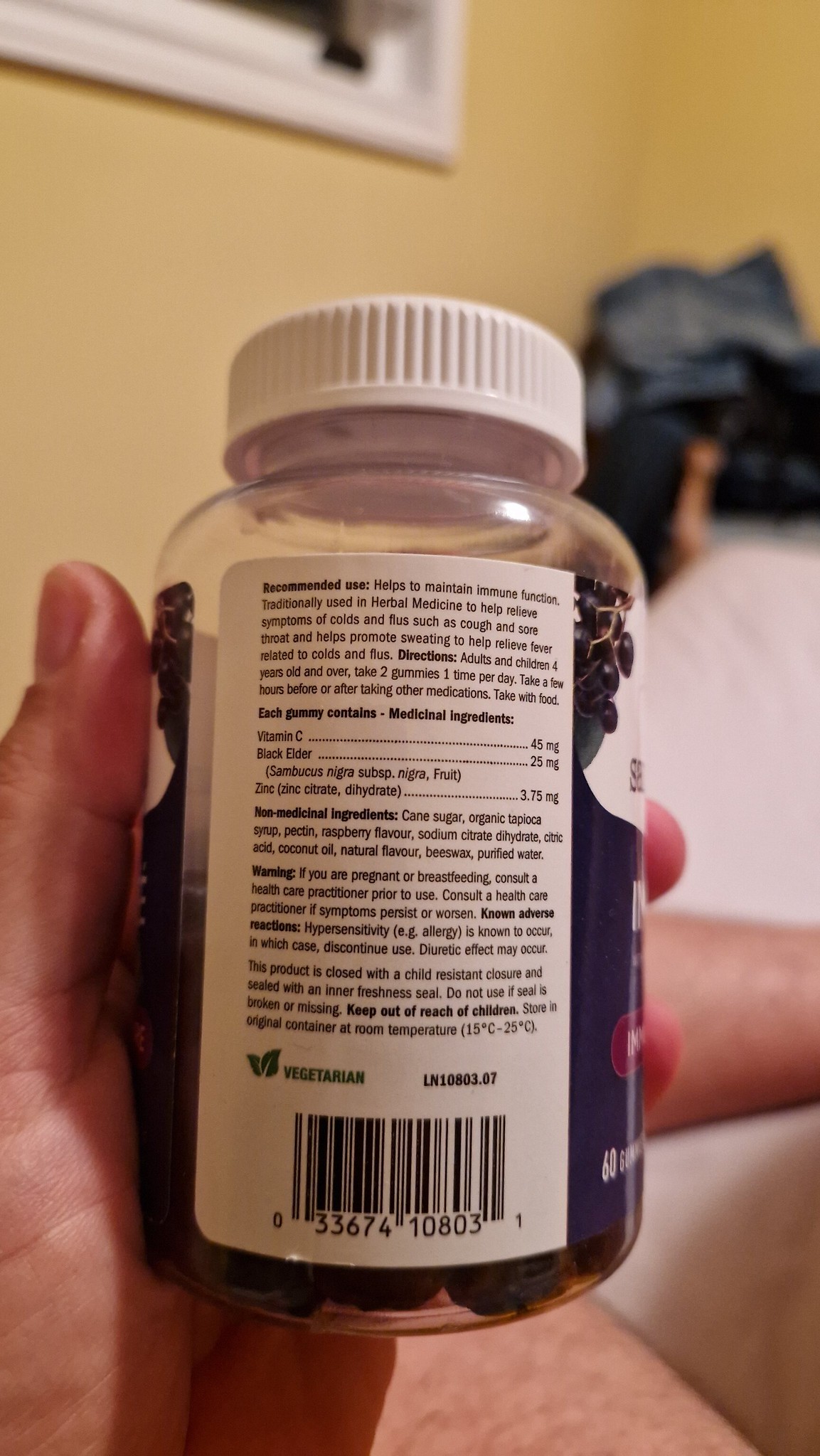In the image, a person is prominently holding a bottle with one hand. The hand is positioned at the bottom left corner of the frame, and part of the person's leg is visible both at the lower edge of the image and through the transparent or partially transparent areas on the back of the bottle. The bottle has a white cap on top and features a detailed label on its side.

The label text, starting from the top left, states: "Recommended use: helps to maintain immune function. Traditionally used in herbal medicine to help relieve symptoms of colds and flus such as cough and sore throat, and helps promote sweating to help relieve fever related to colds and flus." Below that, it provides usage instructions: "Directions: Adults and children 4 years old."